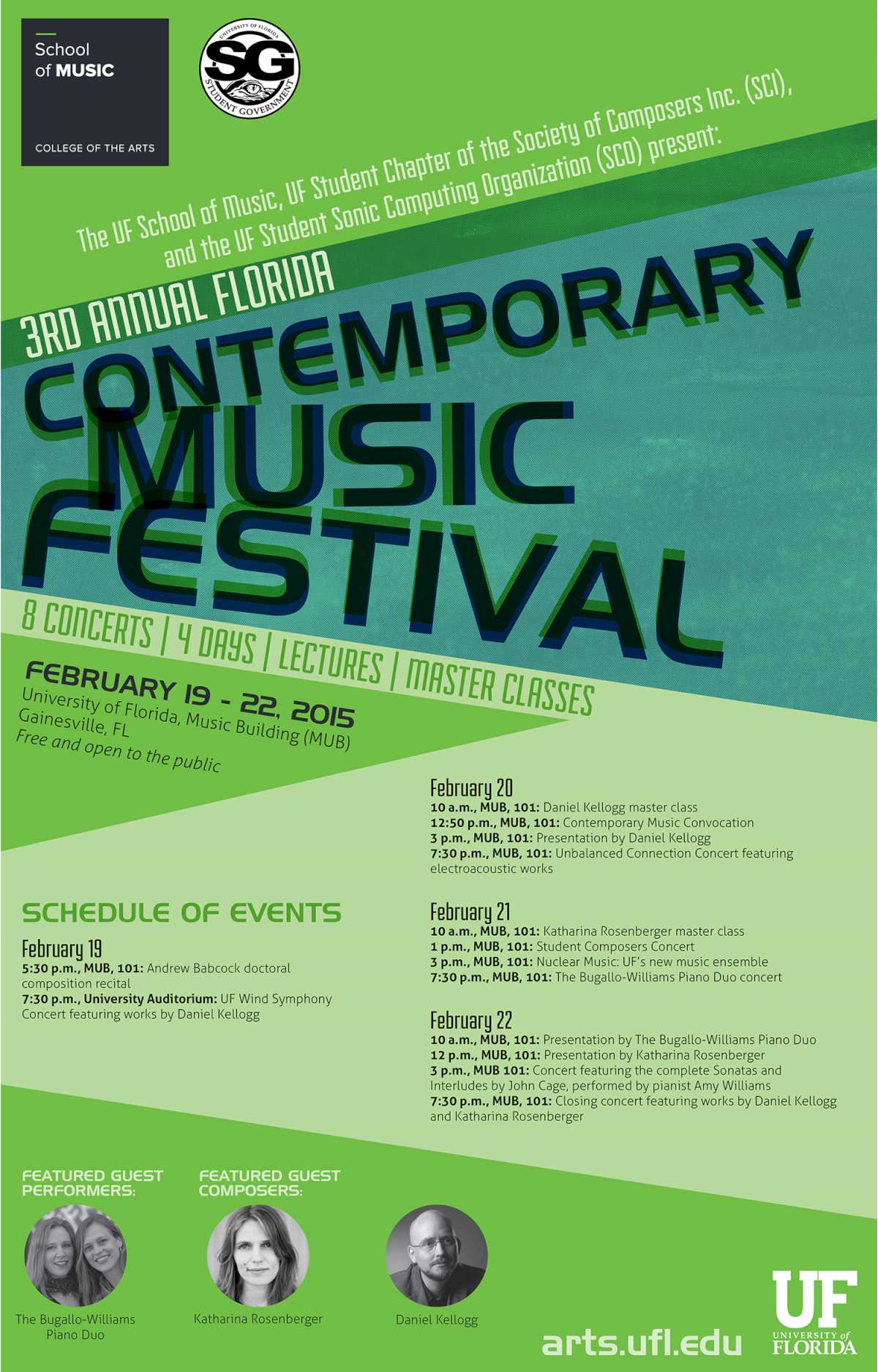A detailed and descriptive caption for the image could be:

---

"The flyer for the 3rd Annual Florida Contemporary Music Festival is prominently designed in white, with key elements highlighted in green. At the top, a gray square features a bow and the letters 'SG' inside a circle, symbolizing the shared effort of various music organizations. The flyer indicates the involvement of the UF School of Music, the UF Student Chapter of the Society of Composers, Inc. (SCI), and the UF Student Sonic Computing Organization (SCL).

The festival is scheduled from February 19-22, 2015, and promises '8 Concerts, 4 Days, Lectures, Master Classes.' Specific time slots for events on February 19th (5:30 p.m. and 7:30 p.m.) are listed, along with additional activities on February 20th and 21st. 

At the bottom, three circles showcase the festival’s featured participants. The first circle contains images of two women under the label 'Featured Guest Performers.' The second circle has a single woman labeled 'Featured Guest Composers.' The third circle displays a man, highlighting another featured guest. 

The flyer also directs interested individuals to arts.ufl.edu for more information."

---

This revised caption carefully details all the elements mentioned in the voice description while maintaining clarity and a structured flow.